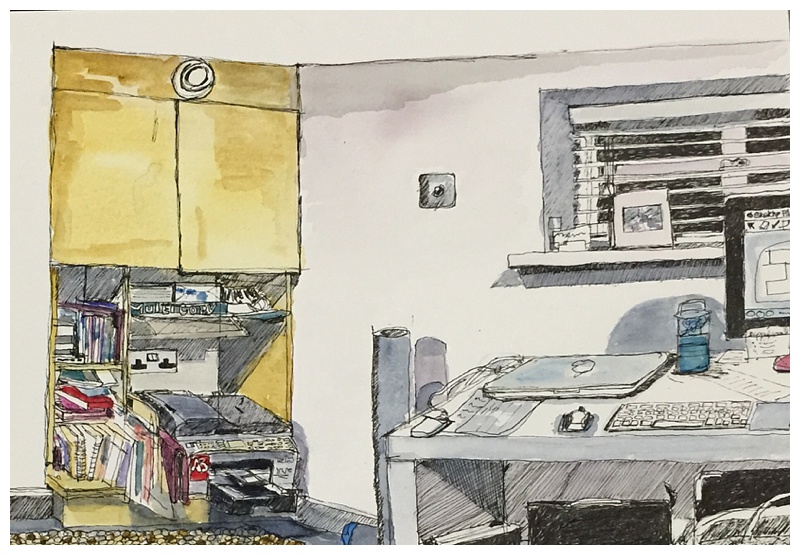This image is an intricate illustration rendered in black pen with a sketchy style and enhanced with watercolour paints. It captures the interior of a minimalist room with white walls, one of which features a light switch. A small, high window adorned with a white slatted blind filters the light, and a photograph sits on the windowsill. 

Central to the scene is a pristine white table, atop which rests a laptop, a computer screen, a keyboard, and various miscellaneous items. To the side, a striking yellow cabinet provides additional storage. The cabinet’s upper half is enclosed by doors, while the open lower half reveals a collection of books. A large printer sits nearby, next to a British-style electrical socket, contributing to the room's functional yet cozy atmosphere.